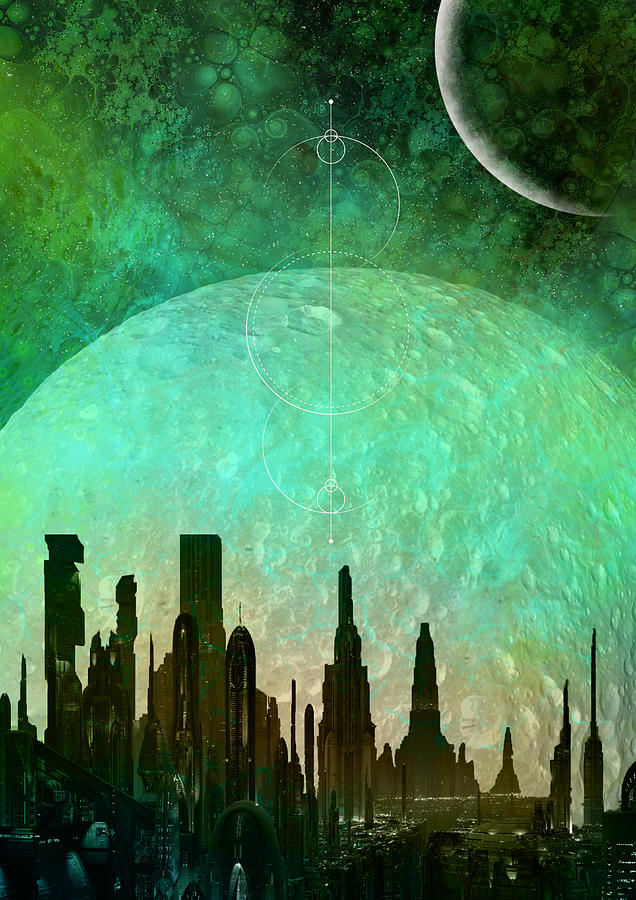The image depicts a captivating piece of science fiction-inspired digital artwork showcasing a futuristic cityscape. At the bottom, a darkened, golden Matrix-style city emerges with towering, sharp-pointed structures of various shapes and sizes, giving an impression of high-tech, modern architecture. Among these buildings, some appear intact while others seem partially demolished, hinting at an underlying narrative of destruction or decay.

Above the cityscape, the background transitions into a space-themed, dark sky filled with intricate green swirls, circles, and splatters that convey an otherworldly aura. Dominating the center is a large, cream-colored orb with hues of blue and green, dotted with crater-like impressions, evoking the image of an otherworldly moon. A distinct vertical white line intersects with three overlapping gold circles, adding to the sci-fi aesthetic.

In the upper right corner, a gray crescent sliver suggests the presence of another planetary body, partially illuminated by a mysterious white light source. The overall composition combines elements of futuristic architecture, cosmic phenomena, and digital artistry, creating a mesmerizing visual narrative.